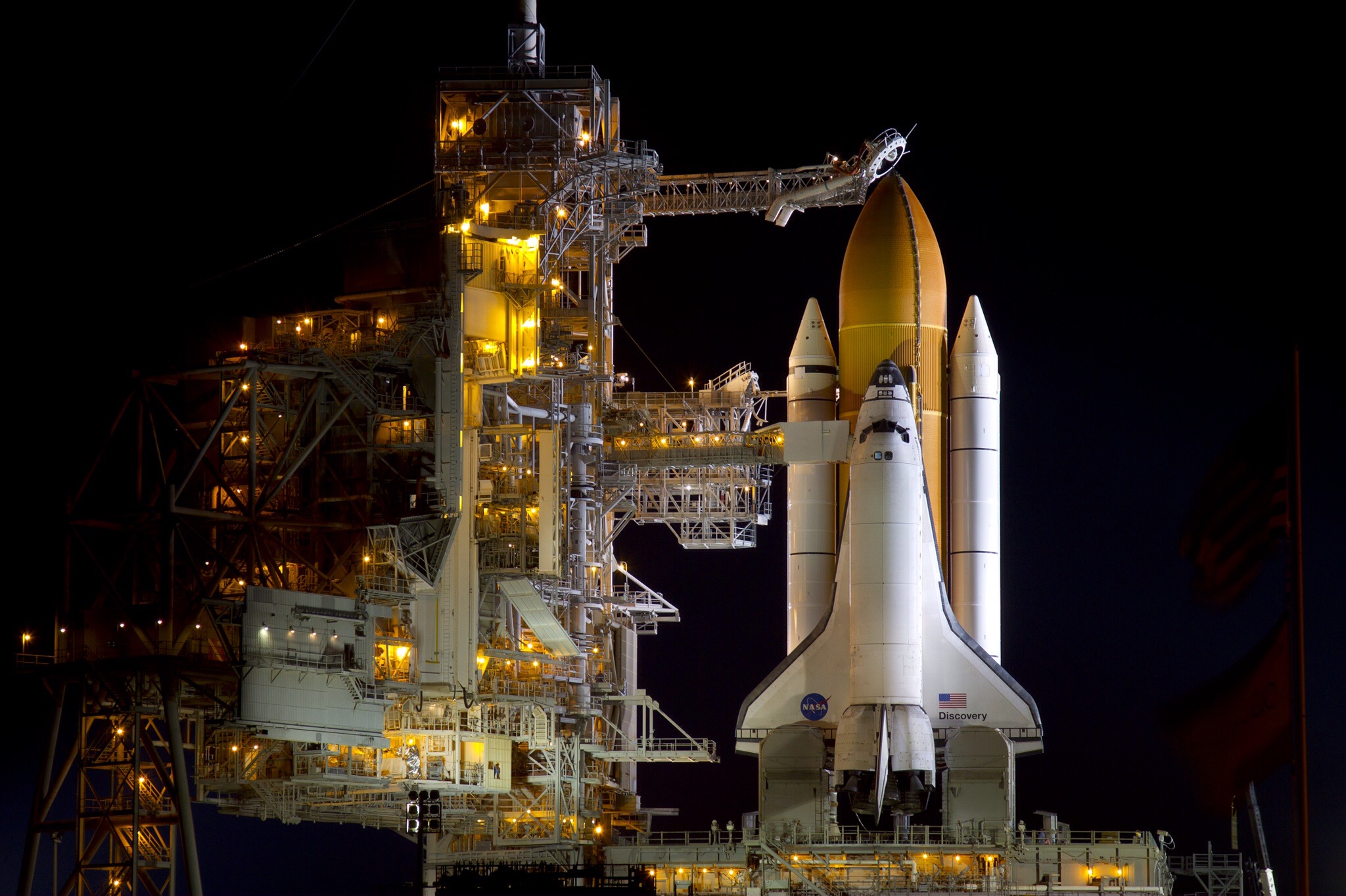Against a stark black nighttime sky, a brightly lit NASA launch site showcases an awe-inspiring space shuttle ready for takeoff. The centerpiece of the image is the towering shuttle, whose white body is sleekly trimmed in black. Prominently displayed on its side are a red, white, and blue American flag and the name "Discovery." On one visible wing, there's a round blue NASA logo beside a small black circle with white writing that's difficult to discern. The space shuttle comprises one large central rocket in an orange hue, flanked by two smaller white rockets. All three rockets are intricately connected to a towering high-rise structure on the left, with multiple gangways and bridges extending from the building to the shuttle, resembling elaborate elevators. This structure and the launch pad beneath are bathed in striking golden-yellow and orange lights, creating a vivid contrast against the dark sky. The launch preparation is meticulous, with the docking station’s detailed safety lights illuminating the complex setup, adding a sense of urgency and readiness to this breathtaking scene.